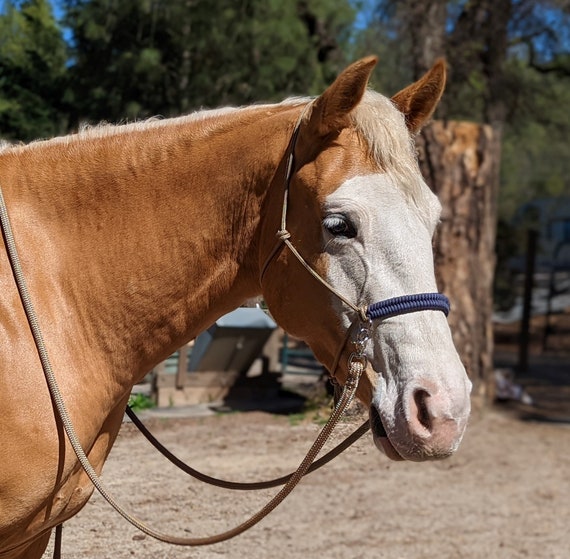This close-up, side-view image showcases the head and neck of a gentle-looking brown horse adorned with a blue and brown muzzle. The horse features a distinctive white face and a light blonde mane, which complements its pale cream muzzle extending from its mouth up to above its eyes. The horse's ears are forward, and its eyelashes mirror the blonde mane. The reins are looped around its neck. In the background, there's clear detail of green trees, suggesting the horse is outdoors. The ground beneath and beyond the horse is gravelly, with the bottom of a small tree and a fence visible to the right. There appears to be a large wooden stump or feeding station present as well. This picturesque scene captures the horse amidst a natural, serene environment.